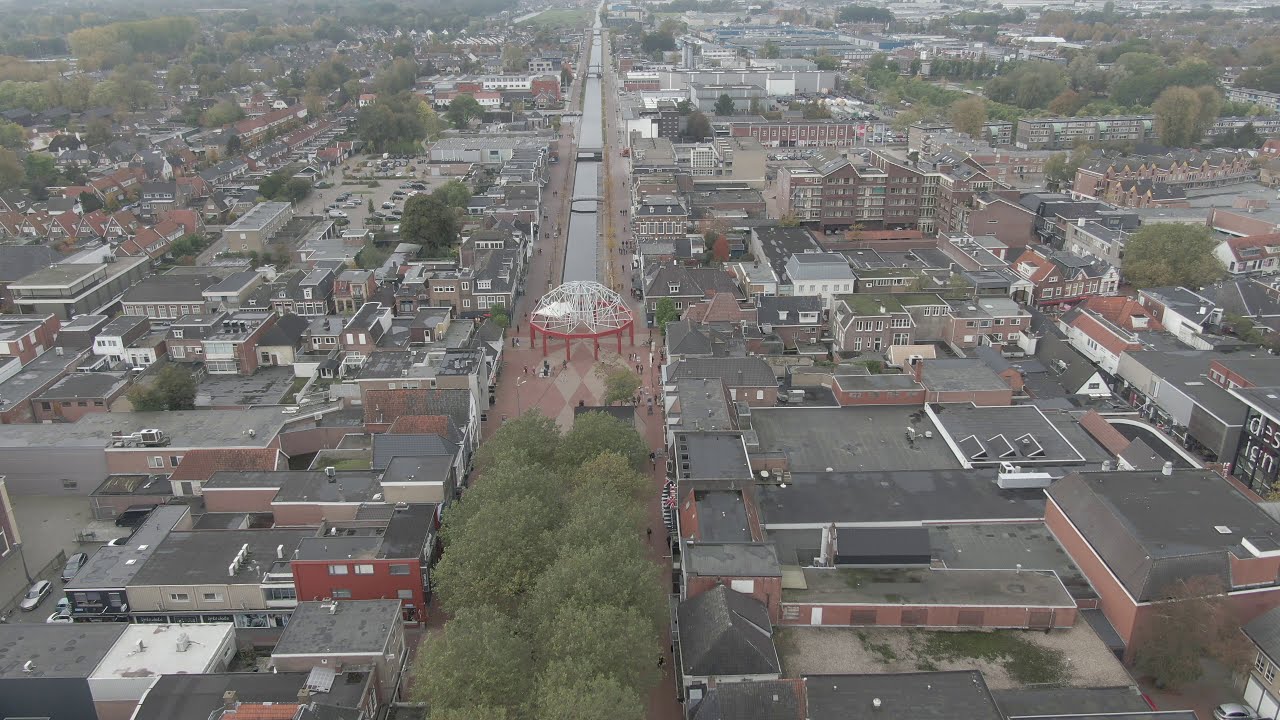This aerial photograph, likely taken by a drone, captures an expansive town, potentially a college campus, with a detailed and vibrant layout. Running vertically through the center is a narrow waterway, evocative of the Washington Monument's reflective strip, crossed by several bridges. On either side of the waterway are broad, tree-lined walkways bustling with people.

In the middle ground of the image stands a striking red and white dome on a platform supported by pillars, adjacent to a courtyard with a red and white checkered walkway filled with visitors. The surrounding architecture includes a mix of older institutional buildings near the center and newer office buildings further out, all with black-roofed structures.

Parking areas are interspersed among the buildings, with numerous cars visible. Trees, both within and outside the building complexes, add to the town's greenery. The scene, captured on an overcast day, features a harmonious blend of nature and urban planning, presenting a vibrant community from a bird’s-eye view.